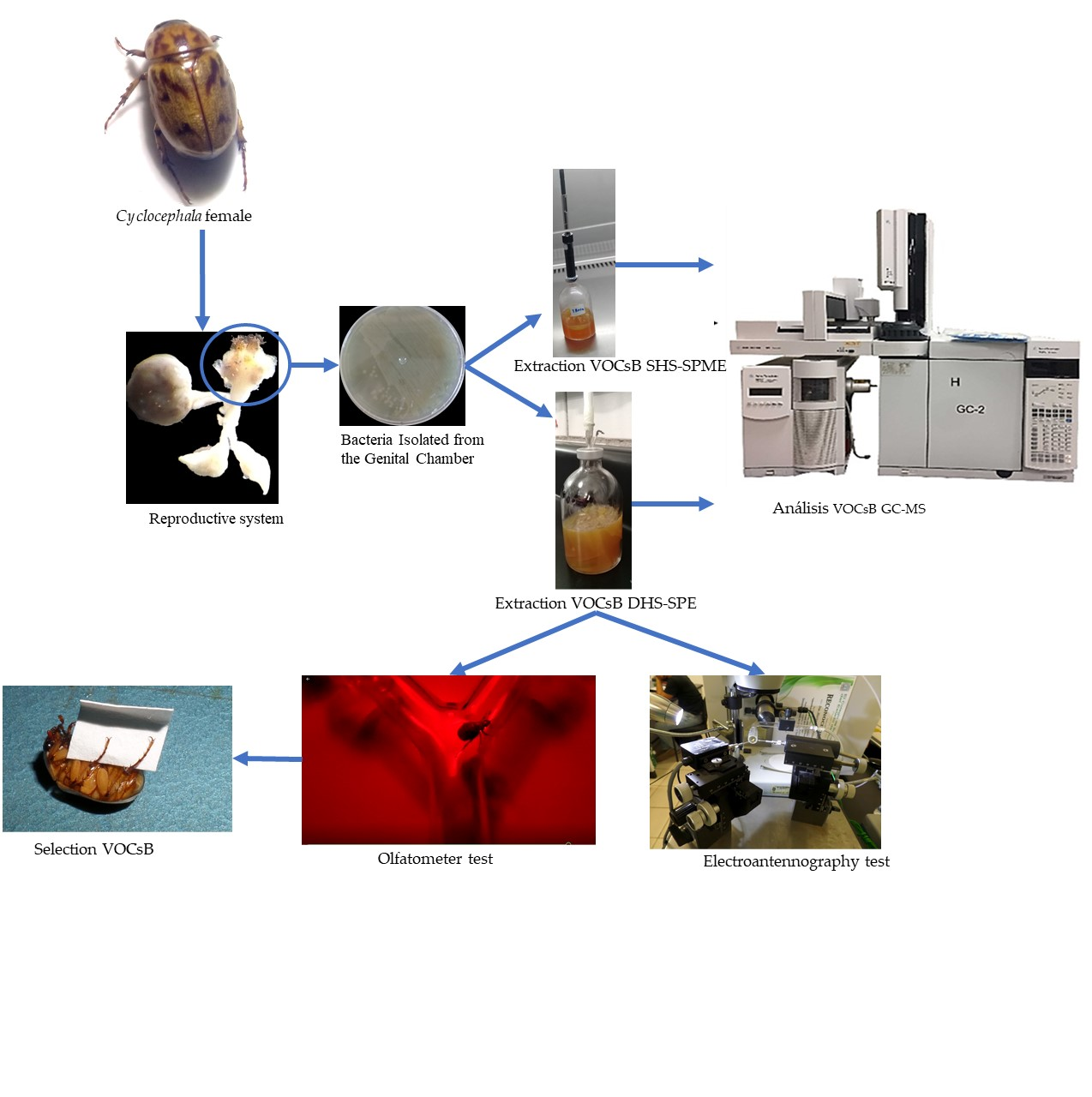This detailed flowchart visually explains the process of analyzing a beetle, specifically labeled as Cyclocephala female, which is beige with light and dark brown spots and squiggles. The flowchart begins in the top left corner with the image of the insect. An arrow points downward to an image labeled "Reproductive System" which displays a small gray egg with white jetting elements tipped in brown. This image has a circled part identifying "bacteria isolated from the genital chamber."

An arrow from the circled bacteria points rightward to two separate extraction processes. The first extraction is labeled "VOC-SB-SHS-SPE" and appears in a clear bottle with orange-brown liquid. The second extraction, labeled "VOC-SB-DHS-SPE," is shown in another clear bottle containing lighter brown liquid. Both bottles are visually indicated to lead into an analysis machine labeled "Analyse VOC-SB-GC-MS," with corresponding arrows funneling into it.

From this analysis machine, two distinct blue arrows indicate further testing processes. One arrow points to an "Electroantennography test" machine, which is depicted with close-up instrumentation and camera-like equipment. The second arrow directs to the "Olfactometer test," showing an image of the beetle in a brightly illuminated red container.

Lastly, an arrow leading from the "Olfactometer test" points to a "Selection VOC-SB" step, which shows the beetle gripping a white piece of paper, positioned on its back against a cyan background. This chart intricately connects each step of the process from the initial identification of the beetle to the final selection phase.